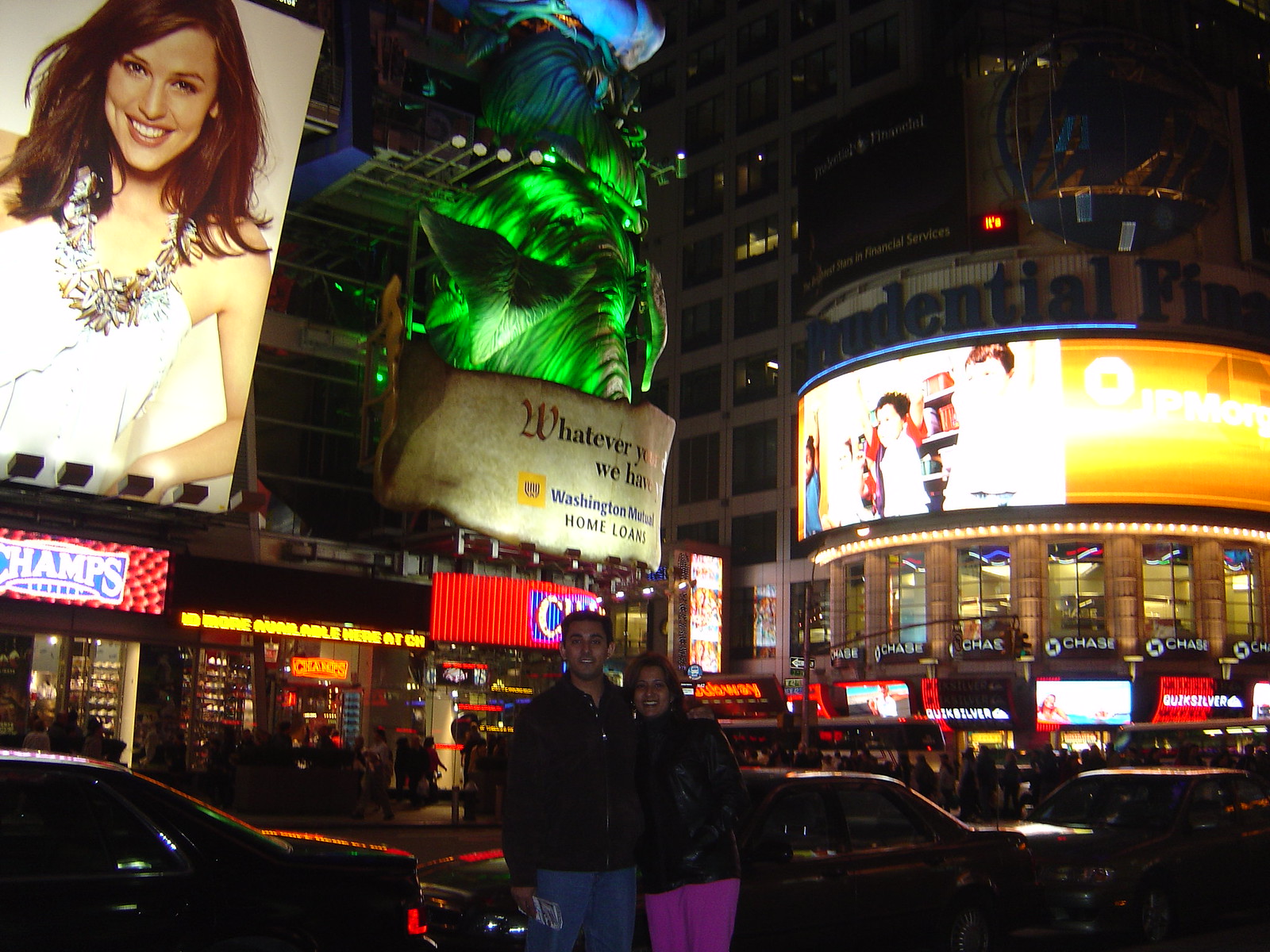In the image, a bustling cityscape at night forms the backdrop, filled with bright billboards, lively traffic, and various advertisements. Dominating the scene are multiple screens and signs, including a prominent billboard on the top left featuring a woman with shoulder-length brown hair, wearing a white dress and a brown lei. To the right of this, a large green display that appears almost plant-like grows out of a sign displaying “Whatever you wish we have it. Washington Mutual Home Loans.”

Further to the right, another screen displays the text "JP Morgan" with a logo featuring a circle within a square and a sign indicating a Chase Bank on a circular building. Below, the words "Prudential Financial" are visible. Amidst this urban landscape, two people are posing for the camera in the foreground—a man on the left and a woman on the right. Both are dressed in black tops; the man is in blue jeans while the woman sports pink or pinkish-purple pants. Cars are parked behind them, and various illuminated signs for businesses, including a Champs store, and possibly casinos, can be seen, enhancing the vibrant, night-time atmosphere of the city square.